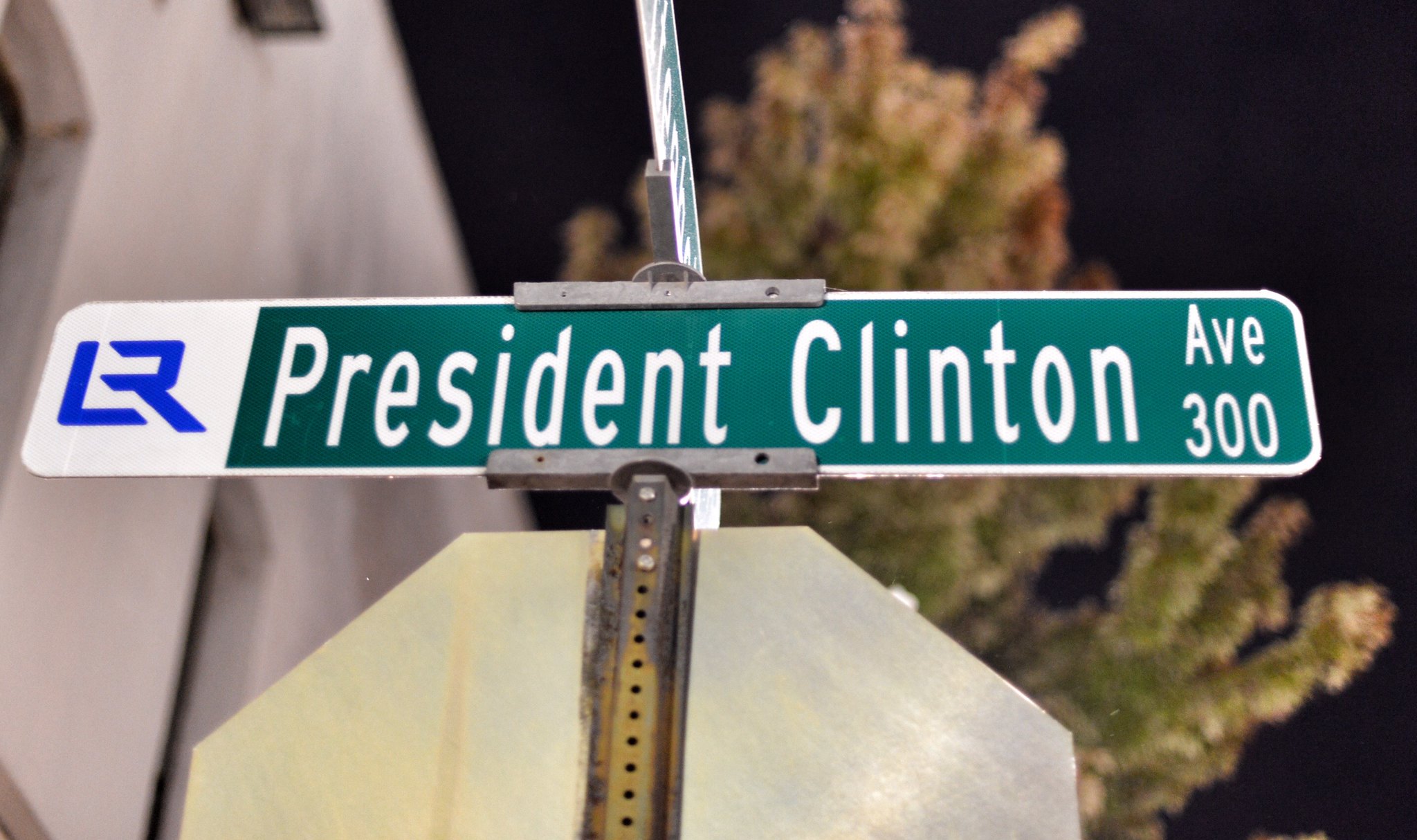This photograph features a close-up shot of a street intersection sign at night. Dominating the frame is the metallic, silver-gray back of a stop sign, with a vertical black metal bar running down the middle. Perched on top of this stop sign is a rectangular green street sign bordered in white. In white lettering, the sign reads "President Clinton Avenue," with the number "300" appearing on the right side. To the left of "President Clinton," a smaller section of the sign features blue lettering against a white background, displaying "LR" or similar characters. In the background, a green tree adds a touch of nature, juxtaposed against a white wall on the left. The sky appears pitch black, indicating it is nighttime. Just below the primary street sign, there's another street sign extending horizontally, but it is partially obscured and unreadable, only showing hints of green and white lettering. The photograph is taken from a slightly low angle, enhancing the perspective from the ground up.